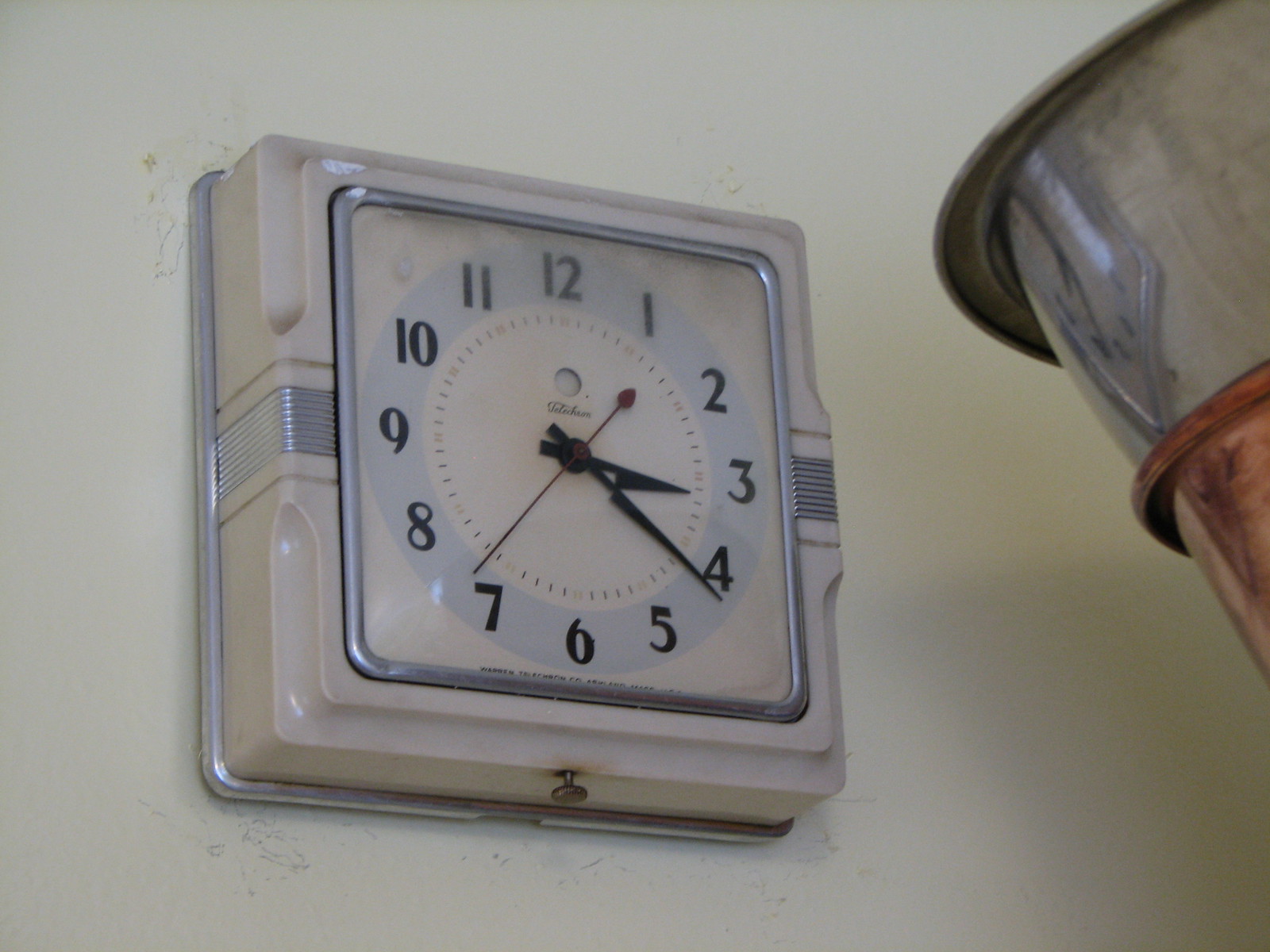This image features a square retro-looking wall clock with notable details. The clock is mounted on a creamy white wall, distinguished by a prominent square silver frame against the wall. The clock itself has a white case with silver ridged sides. The clock face is primarily blue with large, bold black numbers arranged in a circle. Inside this, there’s a white center with black clock hands that point to around 3:21, alongside a notably long red seconds hand. A rusty screw can be seen at the center bottom of the clock's frame.

Additionally, there is a silver band running horizontally from the edges near the 9 and 3 positions, creating a stripe effect. This detail provides an extra layer of contrast against the blue face and white center. Details such as a small hole beneath the number 12 and an unreadable brand name under it can also be observed. The arrangement and structure of the clock, combined with its silver and blue color scheme, provide a vintage aesthetic. To the right of the clock, two vessels, one silver and one copper, are stacked, adding to the scene's ambiance.